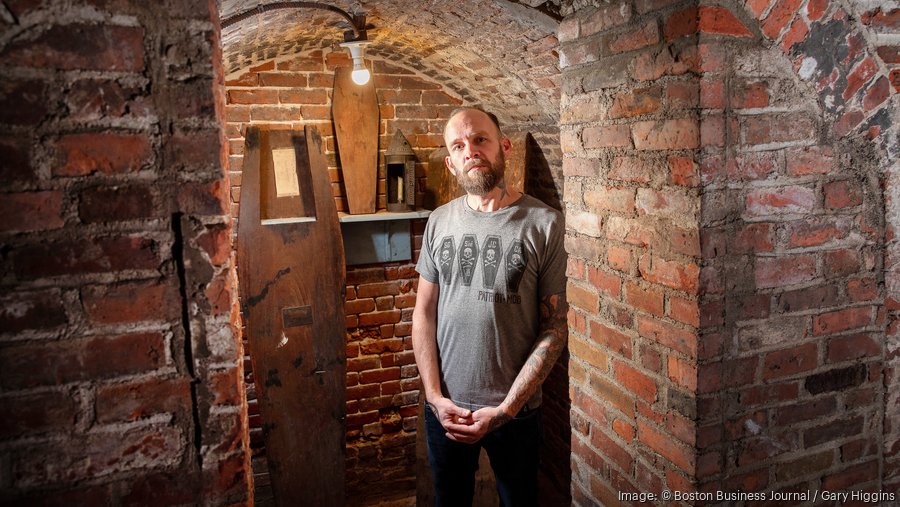In a dimly lit basement room with walls and ceiling made entirely of red brick, a middle-aged, balding man with a dark beard and mustache stands under a single hanging light bulb. The man is wearing a gray t-shirt adorned with four coffin illustrations, each featuring skull and crossbones. To his left, there is a wooden coffin-shaped door with a small window, and on a shelf behind him, there is a smaller coffin-shaped piece of wood along with what appears to be an old-fashioned metal lantern. The image is credited to the Boston Business Journal and photographer Gary Higgins. A mix of red and white bricks adds subtle texture to the room, enhancing the eerie ambiance created by the coffin-shaped objects and the dim lighting.